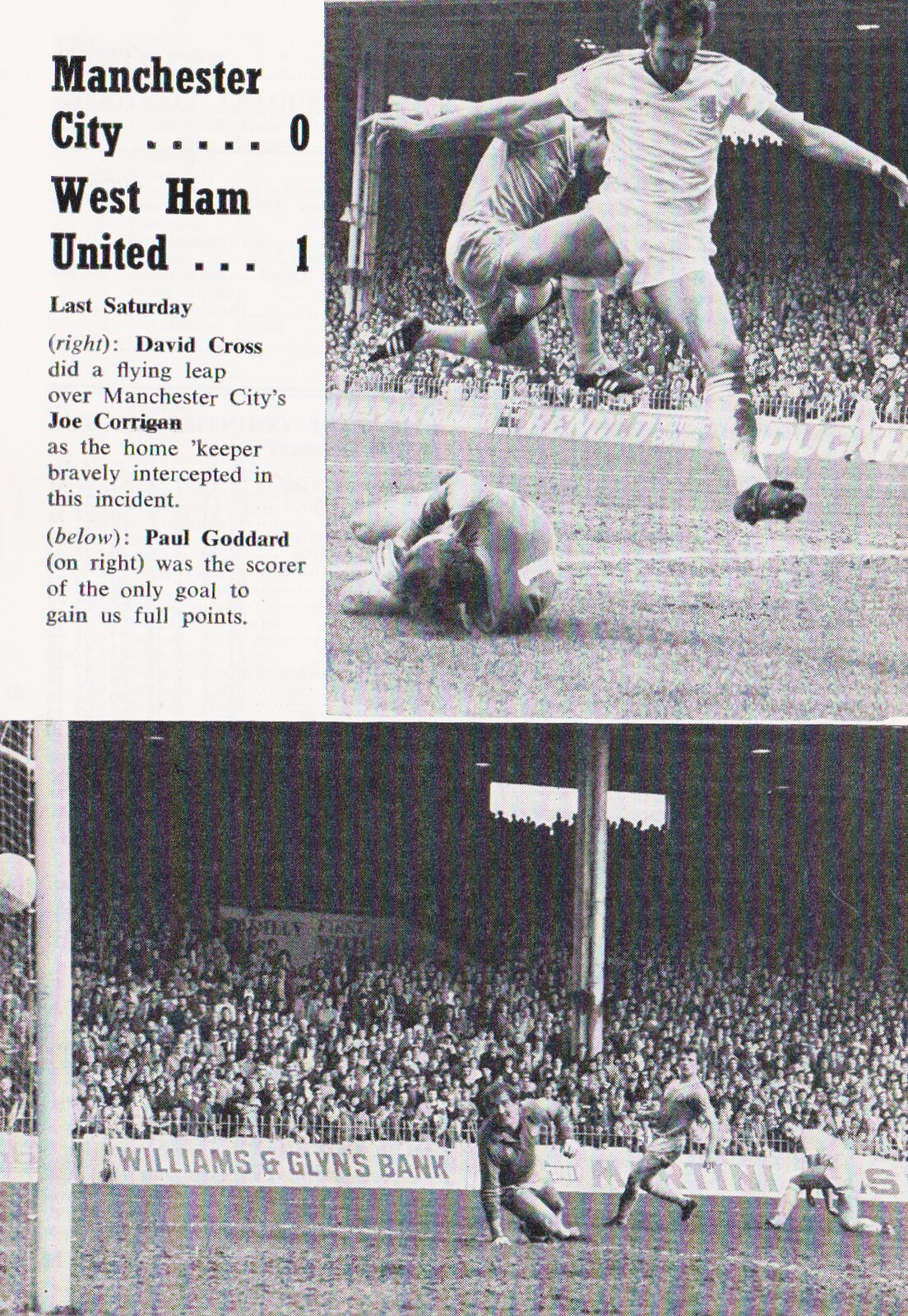This black-and-white image, likely from a vintage magazine or football club program, captures dynamic action from a historic match between Manchester City and West Ham United. The top left features bold text listing the final score: "Manchester City ..... 0 West Ham United ... 1," followed by commentary that indicates the game took place "last Saturday." Detailed narrative below recaps a dramatic moment where West Ham's David Cross executed a flying leap over Manchester City's goalkeeper Joe Corrigan, who was bravely intercepting the ball. Paul Garrard, noted on the right, was the scorer of the match's lone goal, securing four points.

The page is split into two photographs. The upper right photograph, in portrait orientation, vividly shows a soccer player in mid-air with outstretched arms, soaring over another player curled on the ground, while an enthusiastic crowd watches from the stands. The bottom half of the page features a landscape orientation image focusing on the football pitch as the ball makes its way into the goal on the left. Three players, including a goalkeeper, are captured in action with a large stadium crowd in the background. Sponsors such as "William and Glyn's Bank" are visible on the stadium's text.

The photographs and accompanying text, all rendered in vintage print, encapsulate the intense action and atmosphere of this memorable sporting event.